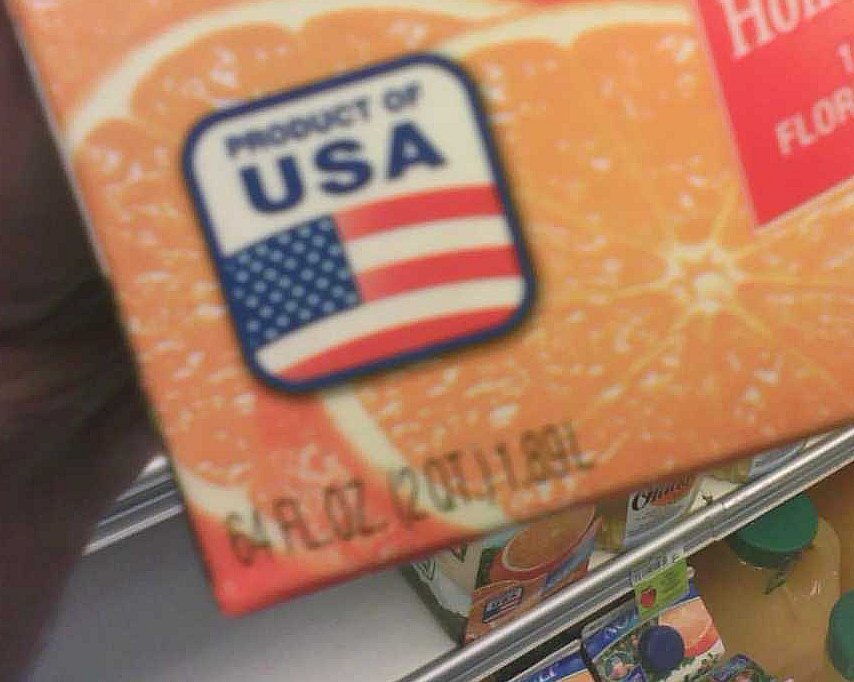A close-up photograph captures the bottom left section of an orange juice carton. Prominently displayed on the front are two overlapping orange slices. Above these slices, a rounded-corner square features the USA flag and the text "Product of USA" in blue, with a blue outline around the square. Directly beneath this logo, the fluid quantity is specified: "64 fluid ounces (2 quarters, 1.89 liters)." The background includes the bottom shelf of a refrigerator or display unit, showing a row of similar orange juice cartons and some lemonade bottles arranged neatly in the corner.